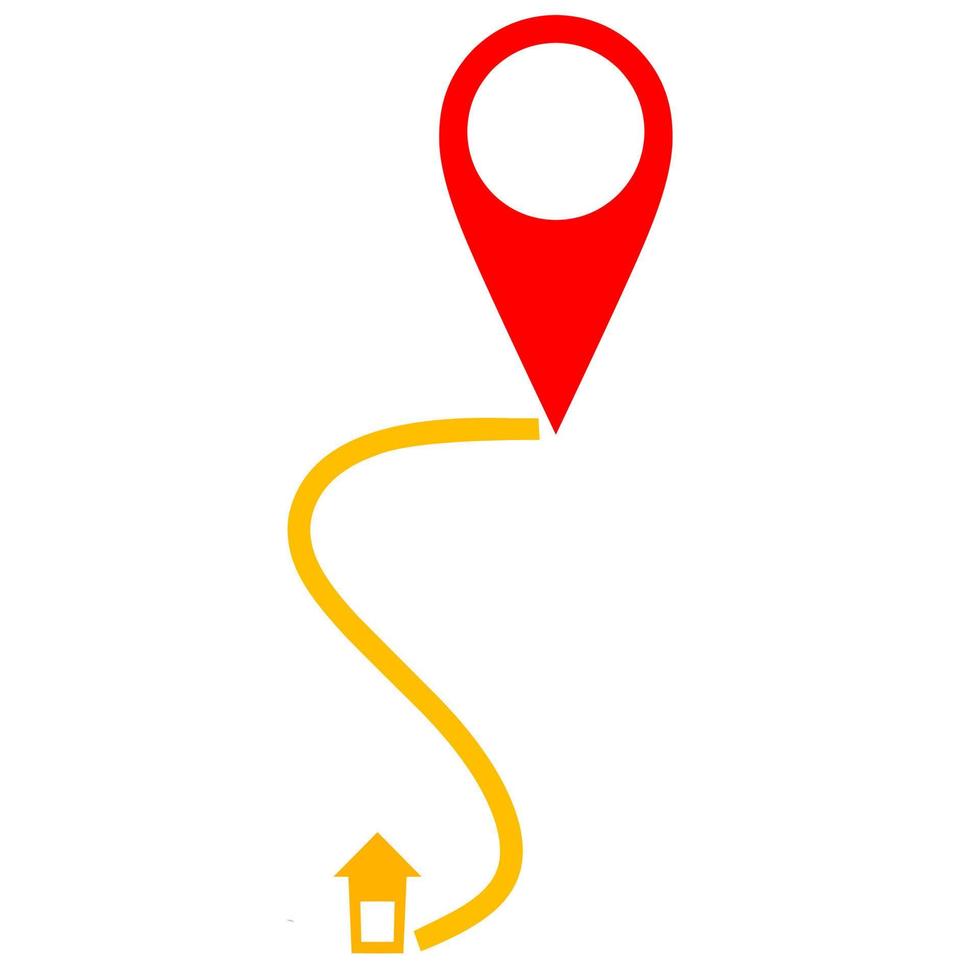This image is a detailed, flat-design illustration featuring a simplified map navigation layout. The background is either white or transparent. At the top of the image, there is a prominent red map pin, shaped like an inverted teardrop with a white circle inside, indicating the current location. A winding yellow line, resembling an S-shape, extends from the pin, moving left, right, and then left again, guiding the viewer towards the bottom of the image. At the end of the yellow line rests a small, stylized yellow house icon with a triangular roof, a rectangular base, and a white square window. This house represents the destination. The color palette is restricted to red and yellow for the icons, enhancing the simplicity and clarity of the navigation theme.